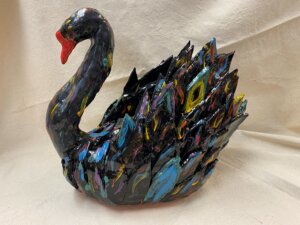This photograph features a detailed, artistic representation of a swan, crafted from what appears to be a combination of glass and ceramic materials. The sculpture captures the left side profile of the swan, with its elegantly curved neck forming an S-shape. The swan's beak is distinctively painted orange, contrasting with the dark, glossy surface of its body. The body of the swan is an intricate mosaic of feathers molded together, displaying an array of reflective colors including dark blue, green, and hints of yellow. The art piece rests on a beige satin-like cloth, enhancing its polished, shiny appearance. The entire setup is positioned near a wall or in the corner, which highlights the reflective properties of both the swan and its background.